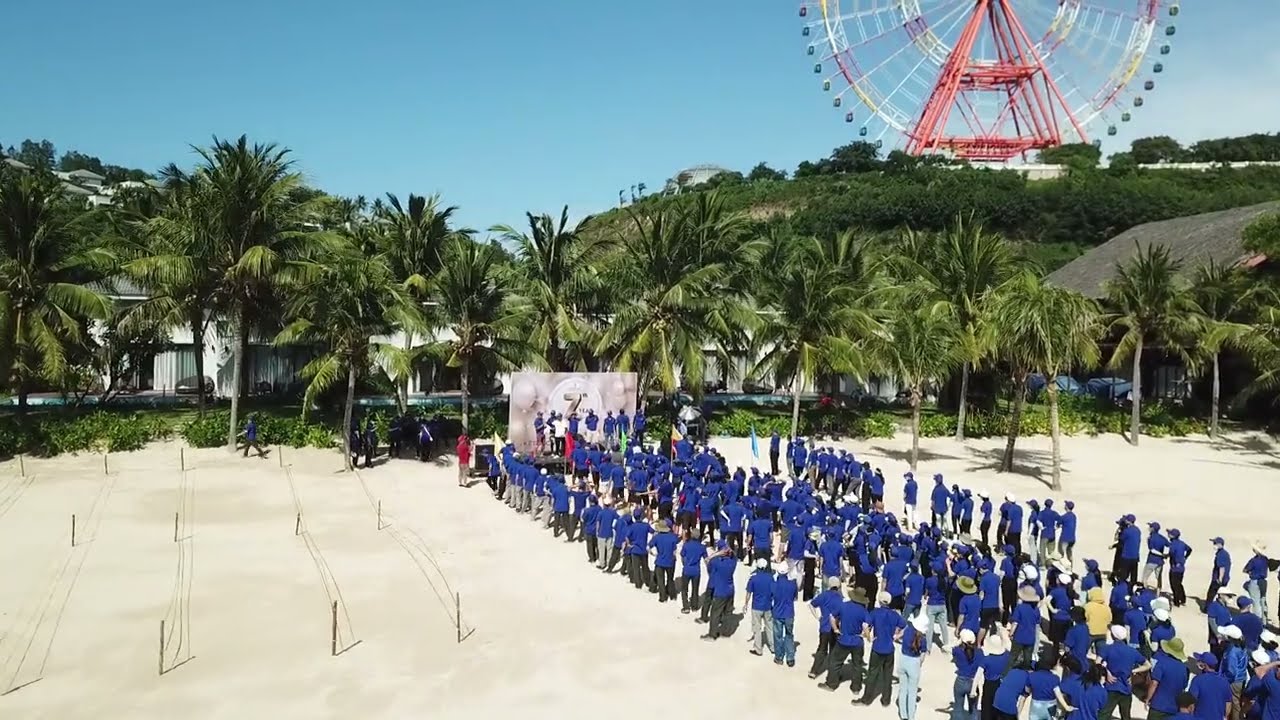In the image, a tropical island setting features numerous green palm trees and a bright blue sky. The foreground shows multiple lines composed of people all wearing identical blue shirts and dark pants, some of them also in white hats. They appear to be waiting for an event or ceremony, as they are all facing towards a stage with individuals similarly dressed in blue uniforms, and one person in a white shirt with black pants. The stage itself has a white background. The scene is set in a sandy area near a structure that resembles an apartment complex, condos, or hotels, likely serving as accommodation for the attendees. Further in the background, there are green hills with the distinctive red and white Ferris wheel standing prominently on the right side of the image. The surrounding environment includes a parking lot area with poles and wires. A striking detail includes a person in a yellow hoodie at the back of the lines and another in a red hoodie walking away from the stage, adding contrast to the otherwise uniform crowd. The overall atmosphere is sunny and festive, suggesting an outdoor event, possibly at an amusement park.